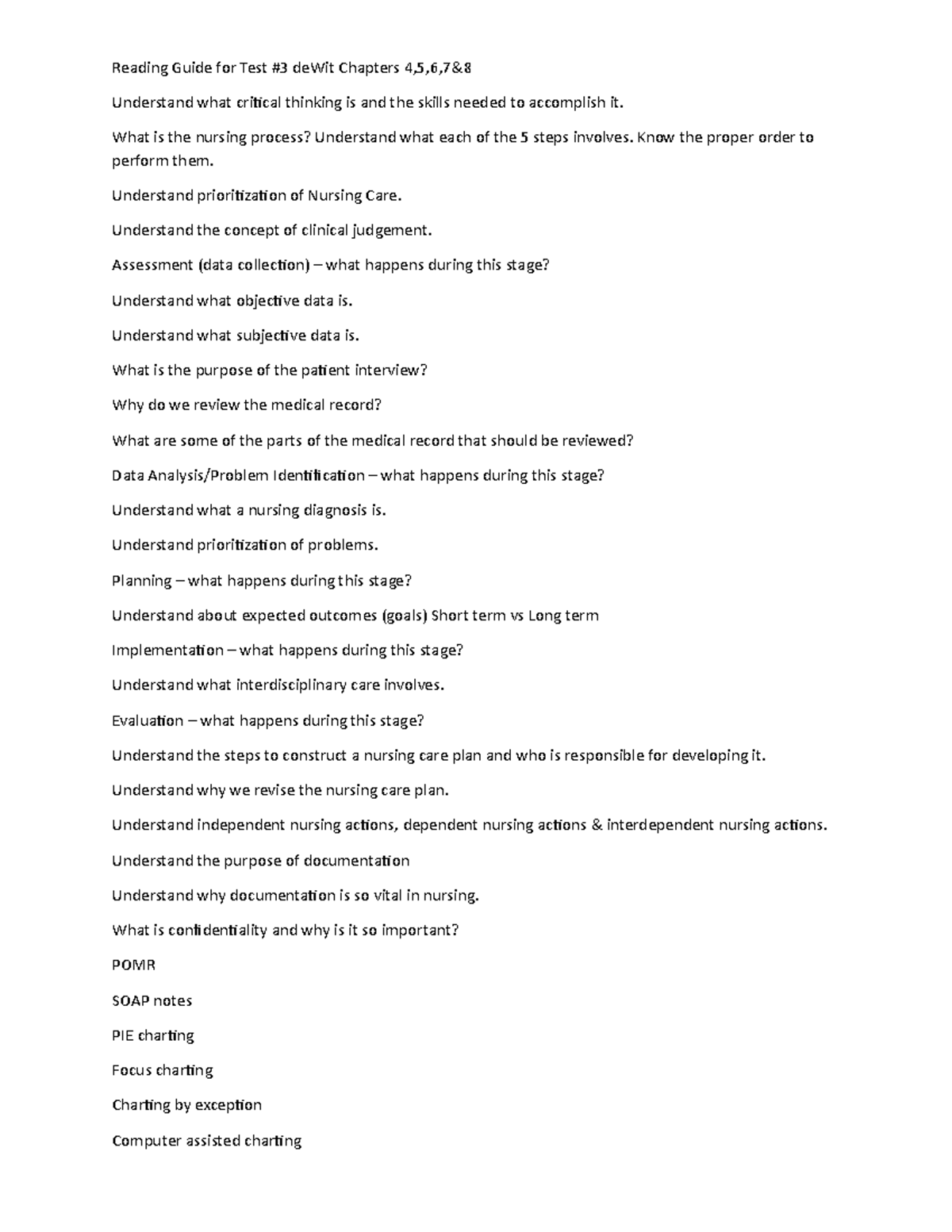**Descriptive Caption:**

This portrait-oriented screenshot captures detailed study notes for Test Number Three in a nursing course. The content, presented in black text on a white background, is left-aligned but not fully visible due to being cut off on the right. It comprehensively outlines key topics and concepts spanning DeWitt chapters 4 through 8, emphasizing critical thinking, the nursing process, and clinical judgment. The breakdown includes:

1. Understanding critical thinking and its necessary skills.
2. The nursing process with a focus on the five steps:
   - **Assessment:** Data collection, objective and subjective data, patient interview, and medical record review.
   - **Data Analysis:** Problem identification and understanding nursing diagnoses.
   - **Planning:** Goals, expected outcomes, and differentiating between short-term and long-term aims.
   - **Implementation:** Interdisciplinary care.
   - **Evaluation:** Steps to construct and revise a nursing care plan, along with understanding independent, dependent, and interdependent nursing actions.

The notes also highlight the purpose and importance of documentation, confidentiality, and various charting methods like POMR, SOAP notes, pie charting, focus charting, and computer-assisted charting. This structurally organized guide aims to prepare nursing students thoroughly for their upcoming test.